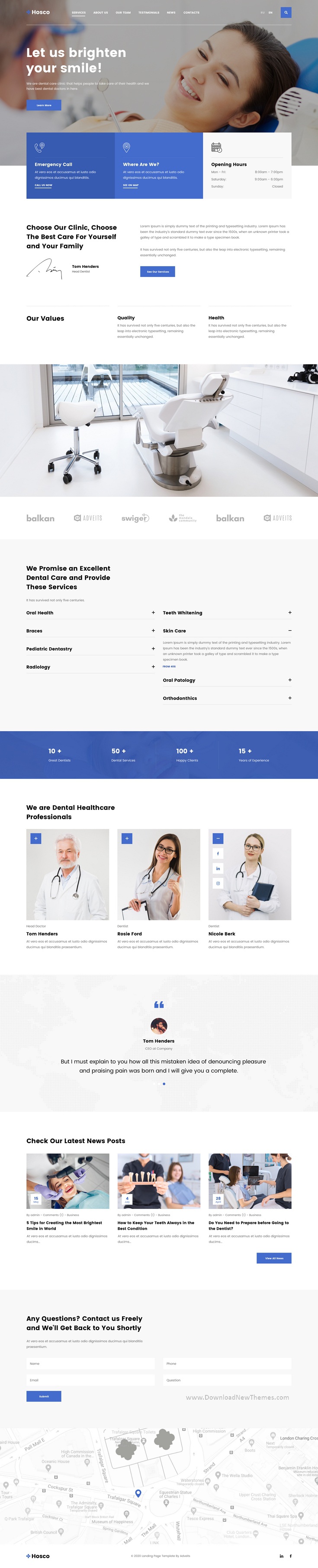The web page opens with a prominent banner at the top, featuring a close-up photograph of a woman reclining in a dentist's chair. Her face is clearly visible, and to the left of the image, a dentist is partially seen in the frame. Superimposed on this picture is the reassuring text: "Let us brighten your smile."

Beneath the header, the layout comprises several rectangular informational boxes. At the very top, there's a sequence of three boxes: dark blue, blue, and white, each containing concise information. Scrolling further down, the page displays another image depicting a typical dental office setting, complete with a patient's chair and a dentist's chair positioned to its left.

Continuing down the page, additional images appear, showcasing individuals who seem to be medical professionals, identifiable by the stethoscopes draped around their necks. These suggest that the website might not be exclusive to dental services but could represent a broader healthcare practice, covering various medical specialties that include both dental care and general medical care provided by doctors.